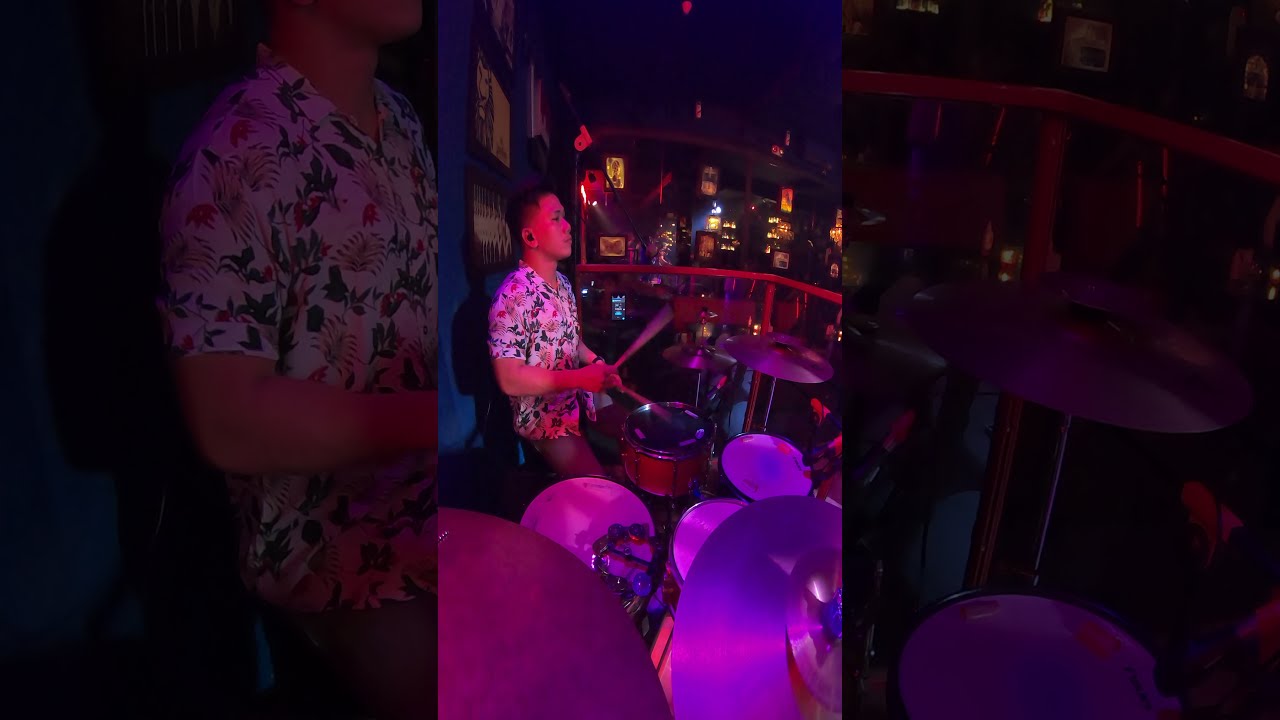In the image, an Asian man is performing on a drum kit in a dimly lit indoor venue. He is seated, facing the right side of the image, and surrounded by a plethora of drums and cymbals. The stage is enclosed by a distinctive red fence. The performer is wearing a white, short-sleeved, button-up shirt adorned with a vibrant floral and leaf print in green and red, accompanied by a black earplug. A purple light casts a glow over the drum set, accentuating the scene. Picture frames can be seen adorning the walls of what appears to be a cozy bar or small venue, defined by blue walls and a shelf that holds several rectangular and square flags.